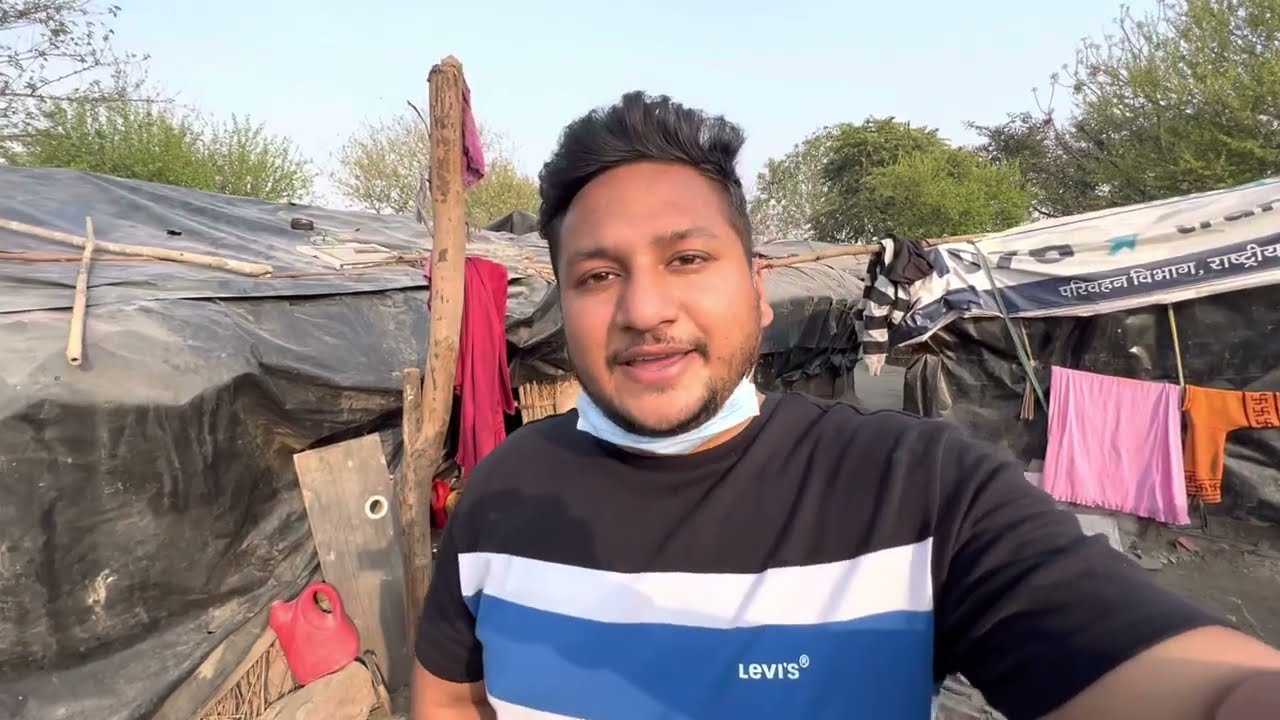In this image, taken outdoors on a clear blue sky day, a man with brown skin, short black hair combed up and back, and a trimmed beard and mustache stands at the center, smiling into the camera while his medical mask rests under his chin. He is dressed in a short-sleeved Levi’s shirt featuring black, blue, and white stripes. Behind him, makeshift structures with roofs improvised from tarps and shopping bags are visible, hinting at shanty-style homes. A clothesline on the right side of the image displays a pink sheet. The background is framed by trees, suggesting a forested area, and there’s also a sign partially visible among the branches, adding to the scene’s rustic and informal ambiance. The overall setting implies an outdoor location in a third-world country.